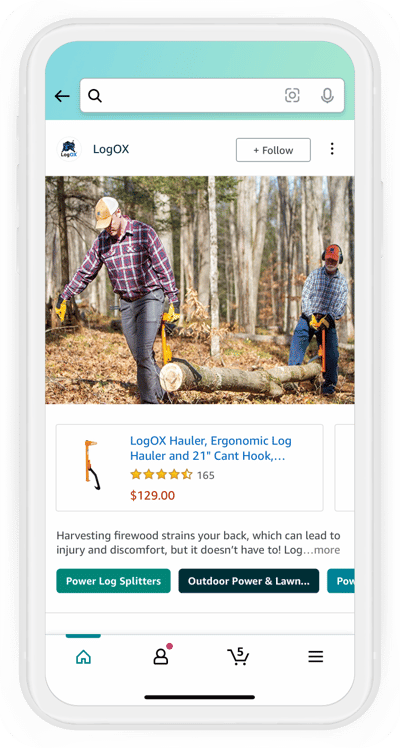A detailed caption for the described image could be:

"A meticulously crafted mock-up displays a white iPhone showcasing a website interface. The screen features a blue header bar at the top, containing a back arrow, a white search field, and options for image and voice search. Central to the header is the 'Log OX' logo, depicting a black and blue bull in an aggressive forward-facing stance. The word 'Log' is rendered in black text, while 'OX' is highlighted in blue. Adjacent to the logo is a 'Follow' button.

Below the header, a vivid image captures two men in a dense forest hauling a massive log using the Log Ox ergonomic log hauler. The men, dressed in trucker hats, plaid shirts, jeans, and yellow gloves, are utilizing a tool with handles painted orange and yellow, indicative of the Log Ox brand. Their determined stance and the hefty log emphasize the product’s utility.

To the left of this scene is a thumbnail image of the Log Ox hauler, accompanied by its product details in blue text on the right: 'Log Ox Hauler: Ergonomic Log Hauler and 21-Inch Cant Hook.' The item boasts a rating of 4-5 stars based on 165 reviews and is priced at $129. A promotional blurb beneath highlights the product's benefits, stating: 'Harvesting firewood strains your back and can lead to injury, but it doesn't have to...'

At the bottom of the screen, navigation options are displayed, including categories like 'Power Log Splitters,' 'Outdoor Power,' 'Lawn,' and another category partially titled 'Power.' The interface concludes with a home button, a user icon, a cart indicator showing five items, and a hamburger menu for additional navigation."